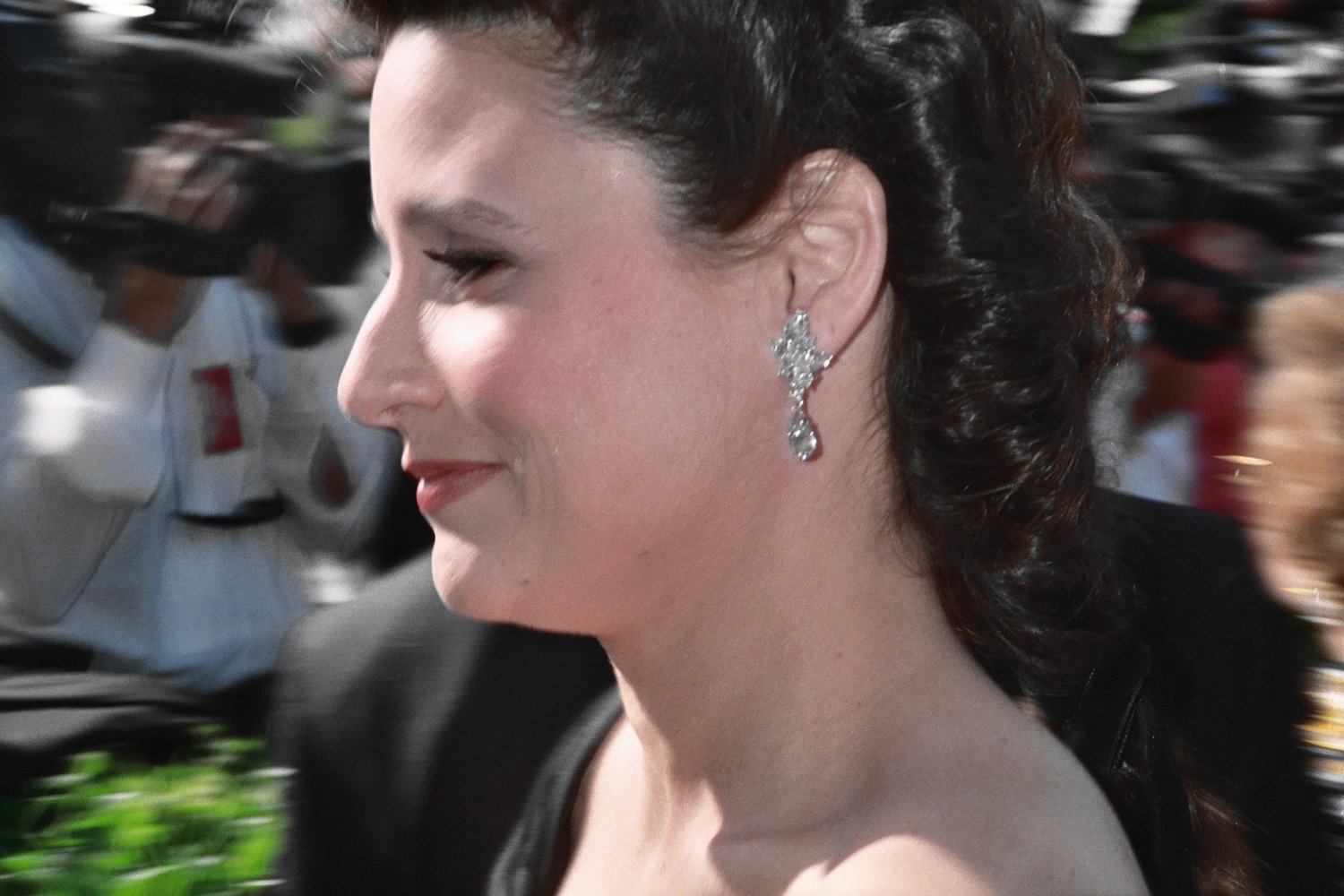The image captures a close-up side profile of a white woman who bears a resemblance to Julia Louis-Dreyfus, although her identity is not confirmed. She has long, dark brown hair and wears a sparkling, dangly diamond earring that catches the light. Her expression hints at a slight smile. She's dressed in an outfit featuring a dark strap over her shoulder, though the exact style is indiscernible. The background, blurred in soft focus, depicts a bustling scene with many people, some of whom are paparazzi or videographers capturing the event. A man in white can be seen with a video camera, filming something beyond her. The bottom left corner of the image shows a patch of green foliage, adding a touch of nature to the otherwise chaotic scene. The overall focus remains sharply on her face, with the surrounding blur emphasizing her presence amidst the crowd.